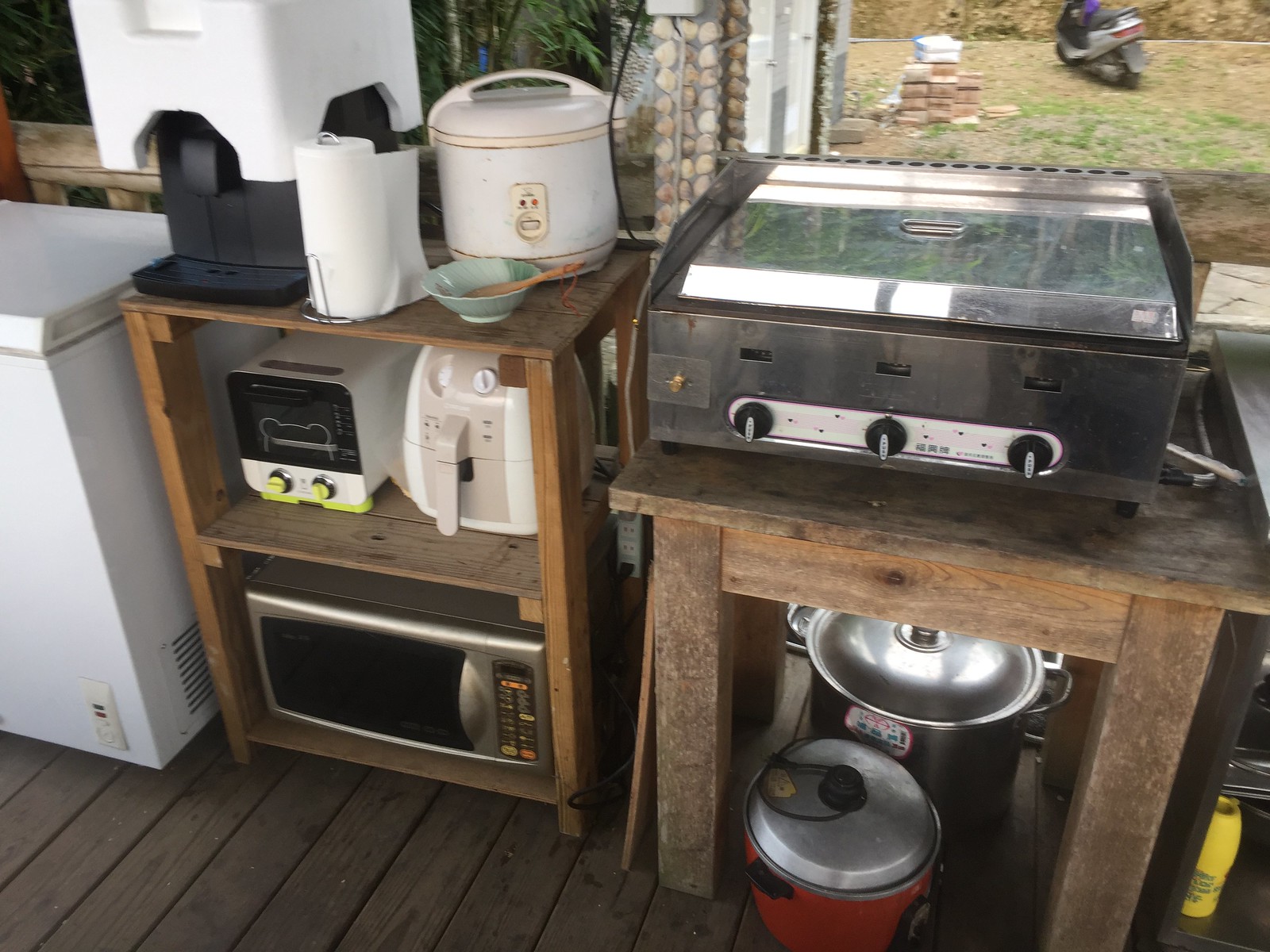This image, taken outside on a wooden deck, captures an elaborate outdoor kitchen setup with a variety of appliances and items. In the foreground, a brown wooden table on the right is adorned with a small grill. Underneath it, there is a large black pot and a smaller red pot. To the left of this table stands another wooden structure that boasts multiple shelves. The bottom shelf houses a microwave, while the middle shelf holds a white air fryer and a toaster oven. The top shelf is cluttered with several items: a white rice cooker, a brown bowl with a wooden spoon, a roll of paper towels, and what looks like an ice machine. Adjacent to this structure is a deep white freezer, partially visible. 

In the upper right corner of the photo, the deck gives way to a lawn that shows signs of wear, with brown patches intermingling with areas of green grass. A black and silver moped, estimated to be around 150 CC, sits on the lawn, adding a touch of motorized convenience to the scene. Behind this array of kitchen equipment, the deck features a charming, log cabin-style railing, offering a rustic backdrop to the modern appliances. The distant view reveals a brown brick house with two white doors, further setting the scene of a well-used, functional outdoor space that bridges the gap between indoor and outdoor living.